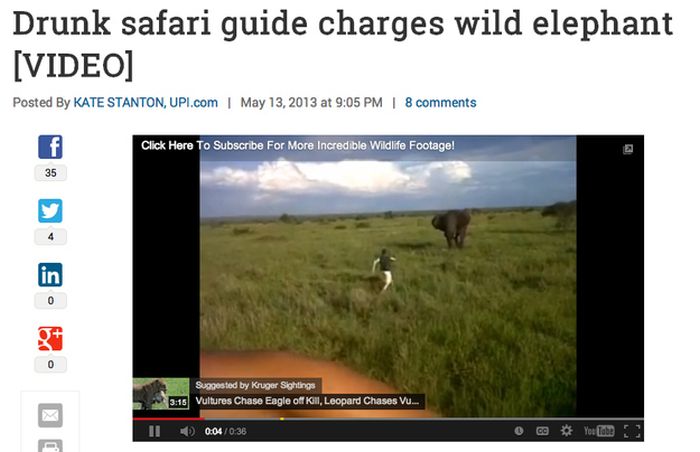The image is a screenshot of a YouTube video titled "Drunk Safari Guide Charges Wild Elephant," posted by Kate Stanton from UPI.com on May 13th, 2013, at 9:05 PM. The video has garnered eight comments. The social media sharing options displayed on the left show the video has been shared 35 times on Facebook, 4 times on Twitter, and has not been shared on LinkedIn or Google+. Additional options to print or email the video are also available.

In the video itself, the caption describes a dramatic scene where a person is seen running towards a wild elephant, with the elephant charging towards the person. A bold text overlay urges viewers to "Click here to subscribe for more incredible wildlife footage!" Beneath the video, a suggested video thumbnail shows a lion with prey in its mouth, titled "Vulture chases eagle off kill, and leopard chases vulture." The duration of the video is 37 seconds, and the screenshot shows it is currently 4 seconds into playing.